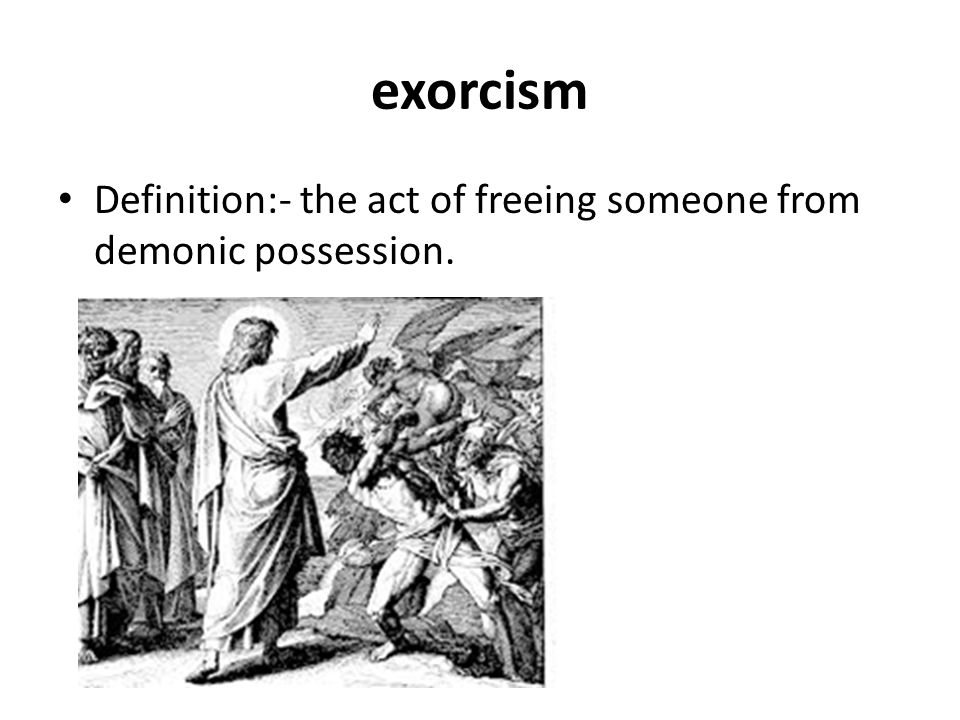The image serves as a detailed illustration of the definition of "exorcism." At the top, the word "exorcism" is presented in bold lowercase letters with the phonetic spelling "e-x-o-r-c-i-s-m." Directly beneath this, a bullet point delineates the definition: "the act of freeing someone from demonic possession."

The central graphic is a black-and-white, grayscale illustration depicting a dramatic, biblical scene. At the heart of the image stands a robed figure, strongly suggested to be Jesus, signified by a radiant halo or sun encircling his head. His right hand is extended outward and upward, fingers pointing to the sky as if to halt the demonic forces before him. To his right, a horde of demonic creatures, including devil's angels and zombie-like beings, writhe and gnash, appearing to advance menacingly.

On the left side of the scene, a group of onlookers — possibly disciples, clad in robes — observe the confrontation with anxious, timid expressions. They appear concerned about the impending conflict and uncertain of the outcome. The overall image is consistent with Christian iconography, emphasizing Jesus' divine authority in warding off evil and protecting the innocent villagers.